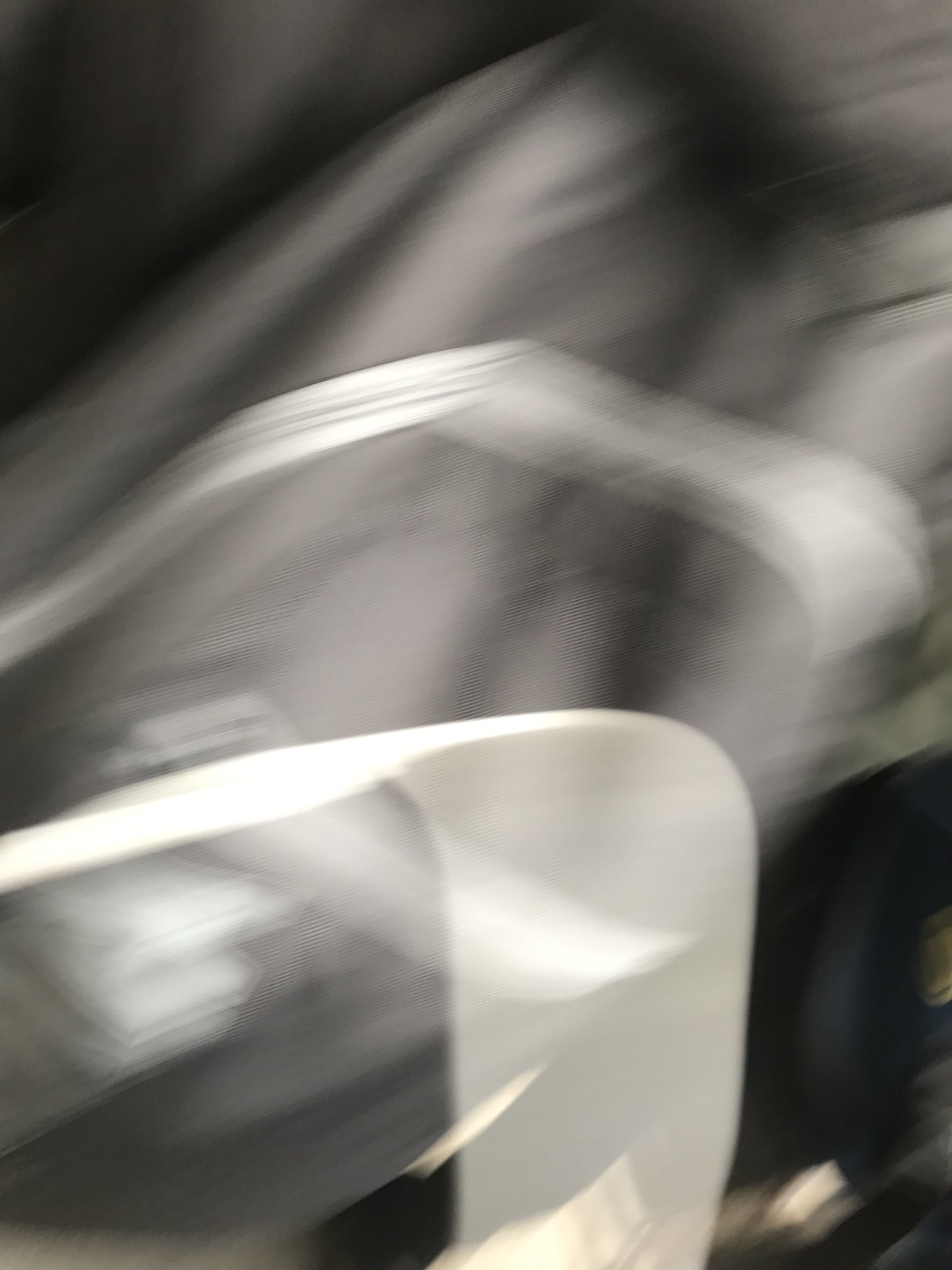The photograph is a close-up, out-of-focus black and white image that appears to capture something in motion, adding to its abstract quality. Dominated by shades of gray and white, the picture features two prominent, thick white ribbons seemingly suspended in mid-air. These ribbons are the most discernible elements against a backdrop that varies from lighter areas to darker corners, especially at the top left and right. The background includes indistinct grayish and white blurred elements, possibly resembling a head or a hand-like device in motion. Additionally, there are hints of sunlight and faint gold reflections towards the lower center, contributing to the overall ethereal and ghostly appearance of the image. The photograph evokes the impression of a spectral figure, or perhaps someone wearing a flowing sheet, adding a haunting, mysterious atmosphere.